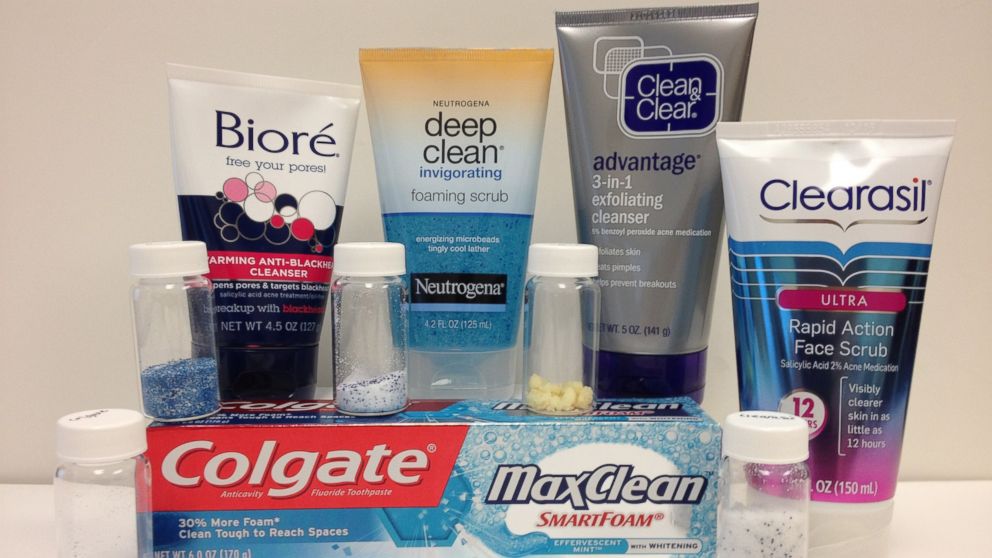This horizontal rectangular image depicts an array of personal care products commonly found in a bathroom, neatly arranged on a clean, white surface against a white background. At the forefront sits a box containing a Colgate MaxClean toothpaste tube, distinguished by its blue color with a red and white Colgate label. The toothpaste is accompanied by various facial cleansers and scrubs in the back, including Clearasil Ultra Face Scrub, Clean and Clear Advantage Exfoliator, Neutrogena Deep Clean Invigorating Cream, and Biore Warming Anti-Blackhead Cleanser. These products come in tubes or bottles of different colors such as white, blue, green, black, orange, and pink. Flanking the toothpaste tube and cleaners are small, clear bottles—one of which appears to be empty and missing a cap that can be seen resting nearby. These items are likely arranged on a vanity countertop, suggesting a typical morning routine setup.